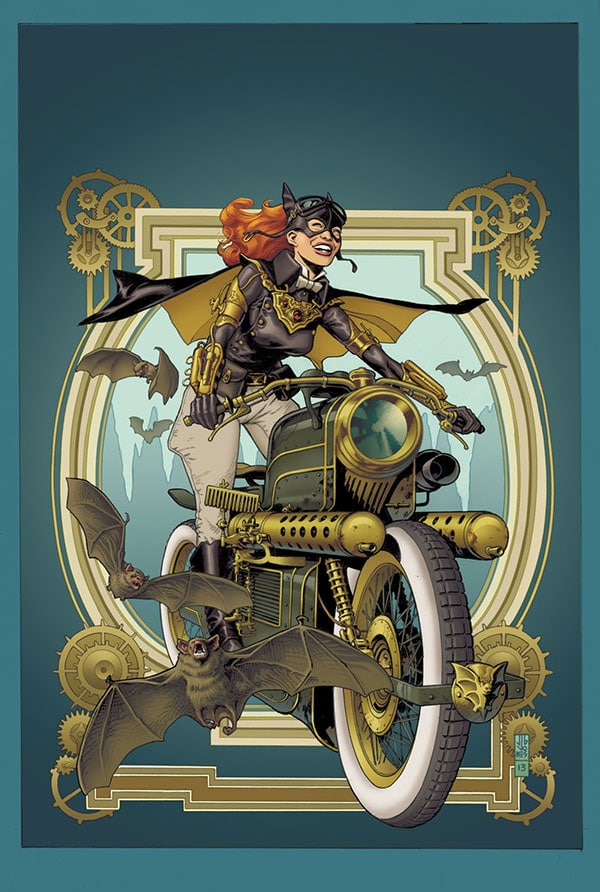The image features a woman dressed in a black leather costume with bat ears and a mask, indicative of a Batman or Batwoman theme. She has long auburn or red hair. She is riding a vintage, steampunk-inspired motorcycle that has a primarily black and gold color scheme, with green accents on the body and gold details on the wheels and handlebars. The background of the image consists of a darker blue inside bordered by a lighter blue frame. There are mechanical gears at the corners of the image, adding to the steampunk style. Bats are flying around the scene, contributing to the eerie and fantastical atmosphere. The entire composition is vertically oriented.